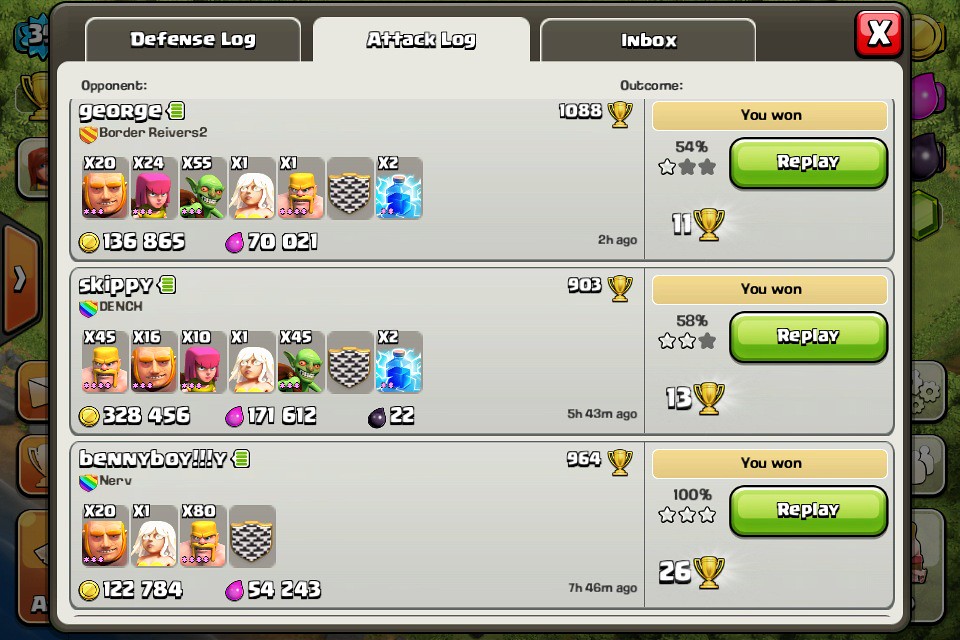This is a detailed color screenshot from a horizontal video game or app, featuring a central panel displaying an "Attack Log." The central panel consists of three tabs labeled in white script: the left tab reads "Defense Log," the center tab "Attack Log" in light gray, and the right tab "Inbox." The "Attack Log" tab is open, revealing a gray panel divided into three sections. Each section lists a player's name in bold white lettering at the top: George occupies the top section, Skippy the middle, and Benny Boy (with three exclamation points and an extra 'Y') the bottom. To the left of each name, an "Opponent:" label identifies the listed players as opponents. On the right side of each section, the outcome of the game is displayed under a winning statistics column labeled "Outcome." Each section includes a green "Replay" button and a trophy icon at the bottom left, which indicates the points assigned to each player, with a "You won" heading in cream and black text above the button. The design and elements are typical of a video game interface, demonstrating a focus on tracking and reviewing gameplay outcomes.